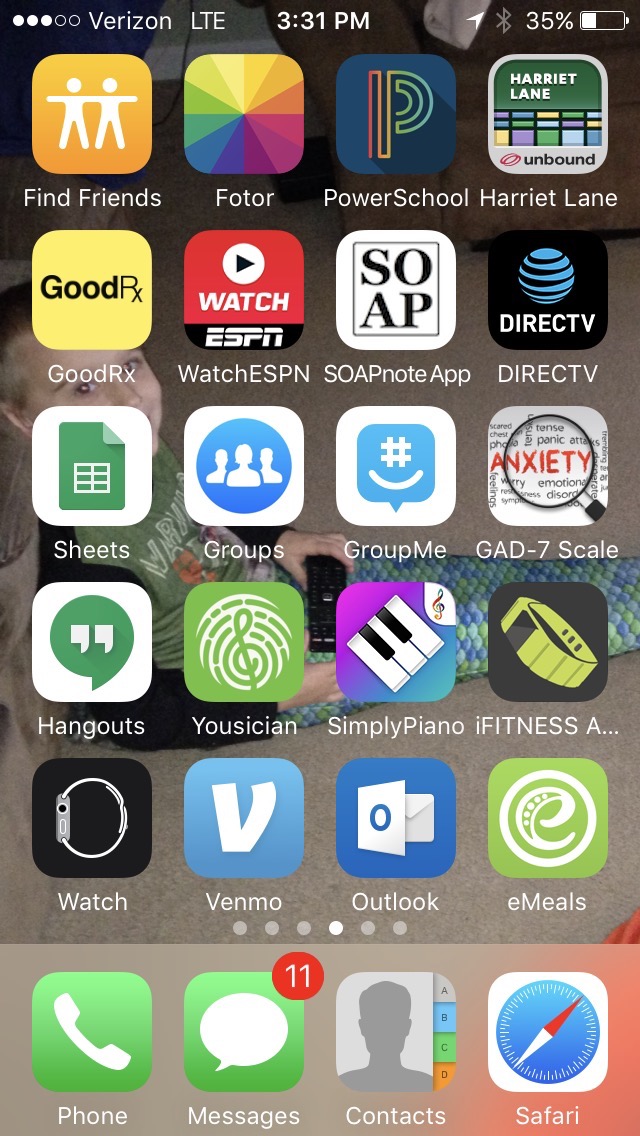The image is a vertically-oriented rectangle, appearing to be a screenshot taken from an iPhone. At the very top, a series of white and blank circles indicate multiple app pages. The status bar reads "Verizon LTE 3:31 PM" and features icons on the right: an upward-pointing arrow, a Bluetooth symbol, and a battery indicator showing 35%.

The main section of the screenshot displays 20 apps, while the dock at the bottom contains four more. The background image is of a young boy sitting on a couch, holding a remote control.

The dock includes the apps: Phone, Messages (with 11 unread messages), Contacts, and Safari. The main apps visible on this page are:

1. Watch
2. Venmo
3. Outlook
4. Emails
5. iFitness
6. Simply Piano
7. Musician
8. Hangouts
9. Sheets
10. Groups
11. GroupMe
12. GAD7 Scale
13. DirecTV
14. Soap
15. Note
16. App
17. Watch ESPN
18. GoodRx
19. FindFriends
20. Photor
21. PowerSchool
22. Harriet Lane

Additionally, there are dots indicating this is one of six pages of applications.